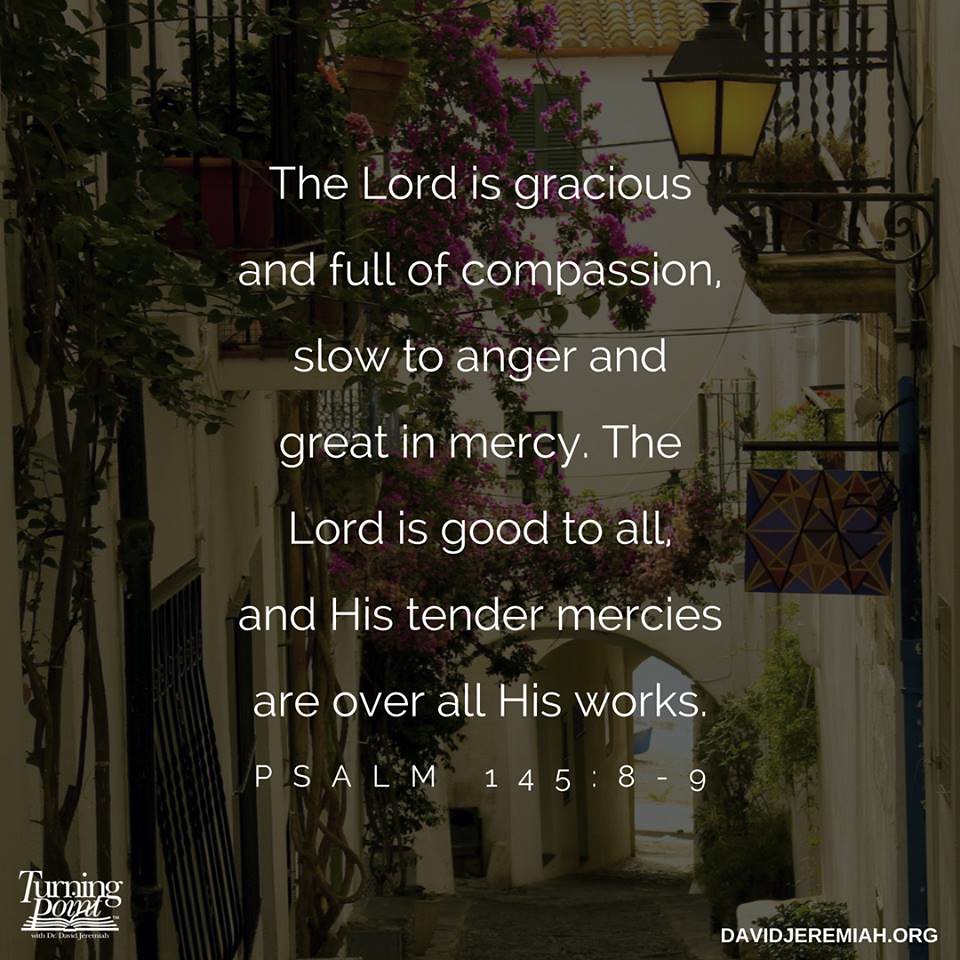The image depicts a serene and picturesque scene of a quaint, digitally-rendered courtyard framed by charming buildings. The background features a three-story house adorned with several balconies, all intertwined with lush greenery, including a tree, bushes, and vivid pink flowers. The architectural details, although slightly blurred, showcase elegant design elements such as a street light and a lamp hanging from one of the walls. At the forefront, there is a house with a prominent roof leading into the scene. An archway under which a street extends can also be seen, adding depth to the composition.

Centrally placed in the image, white text delivers a soothing biblical quote: "The Lord is gracious and full of compassion, slow to anger and great in mercy. The Lord is good to all, and His tender mercies are over all His works." (Psalm 145: 8-9). In the bottom left corner, the logo "Turning Point" accompanied by an image of an open book and the name "David Jeremiah" is displayed. On the bottom right corner, the website "davidjeremiah.org" is visible, anchoring the inspirational message.